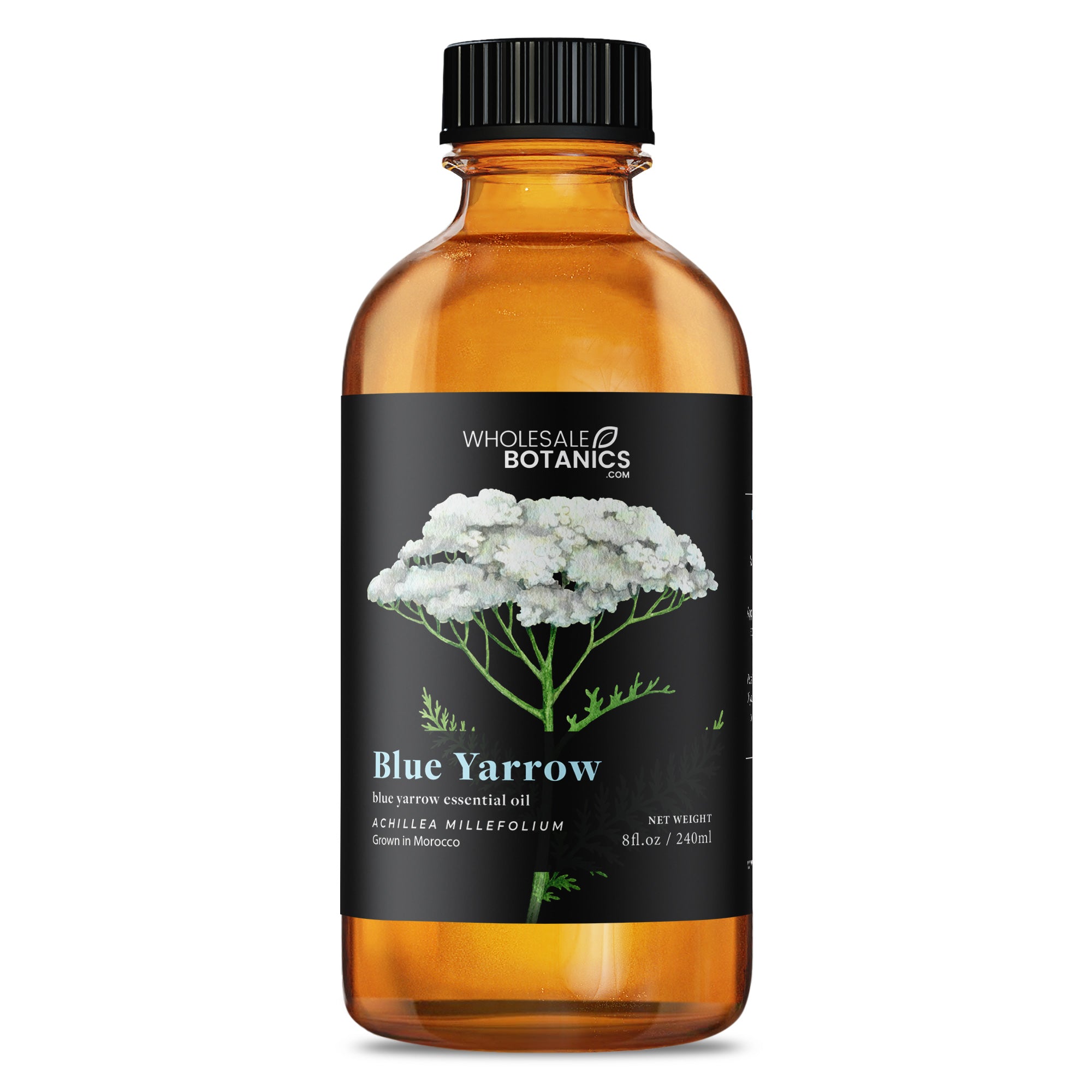The image features a brown bottle of Blue Yarrow Essential Oil from wholesalebotanics.com. The bottle, which has a capacity of 8 fluid ounces (240 milliliters), is capped with a black, ridged twist-off cap. The label, predominantly black, covers two-thirds of the bottle and includes detailed information about the product. At the top of the label, the brand name Wholesale Botanics is displayed in white lettering. Centered on the label is an illustration of a yarrow plant with green leaves and white flowers. The Latin name of the plant is also included but not specified here. Below the illustration, in blue lettering, it reads "Blue Yarrow Essential Oil." At the bottom left of the label, it states the net weight of the bottle as 8 fluid ounces (240 milliliters). The essential oil is noted to be grown in Morocco. The background of the image is stark white, designed to draw attention to the product’s minimalistic and straightforward presentation. The bottle’s function and appearance align with typical essential oils, focusing on essential details and a clean, professional look.